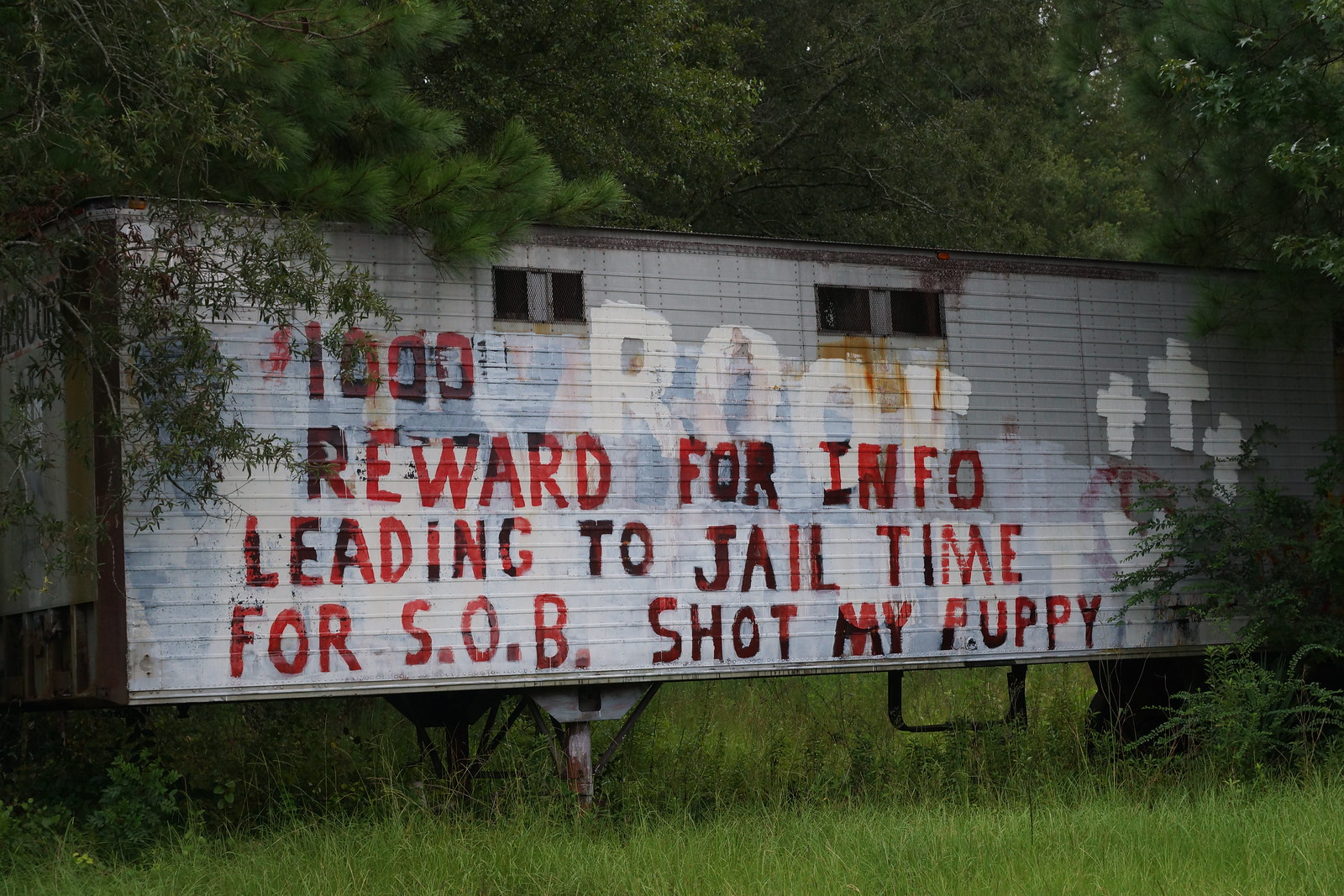In this photograph, there's an old, long, and rectangular white trailer, heavily rusted and seemingly abandoned. The trailer is surrounded by tall green grass and dense tree branches, with leaves encasing it from the top and sides, creating a sense of seclusion. The side of the trailer is marred by multiple spray-painted messages. In bold red letters, it states: "$1,000 REWARD FOR INFO LEADING TO JAIL TIME FOR S.O.B. SHOT MY PUPPY." Nearby, the word "ROOF" or "ROOT" is roughly painted in white letters. Additionally, three prominent white block crosses are positioned on the upper right side of the trailer. Rectangular black vents are visible along the side, and the trailer is elevated on rusted legs, hinting at years of neglect. The overall scene conveys an eerie, deserted atmosphere, amplified by the encroaching nature that threatens to completely consume the trailer over time.